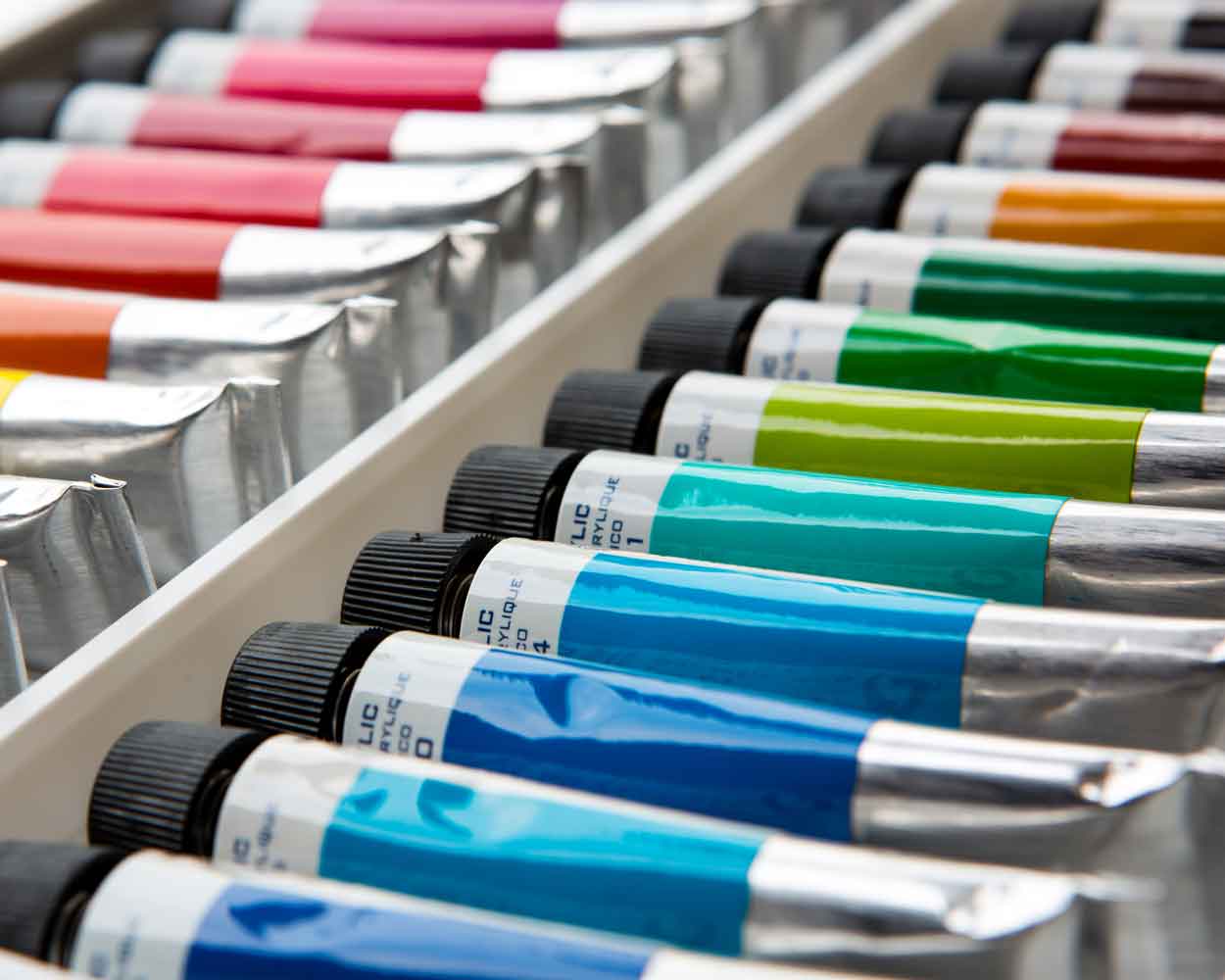The image is a close-up photograph of neatly arranged acrylic paint tubes within a white compartment, possibly a drawer or shelving unit. The tubes have silver bodies with black caps and a small section displaying the color inside. There are two rows of these tubes separated by a white divider. The prominent front row displays an array of colors transitioning from various shades of blue to aqua, green, orange, red, brown, and finally black, although the background is slightly blurry due to the depth of field. The less prominent back row features tubes that transition from yellow to orange, a blood orange, different shades of pink, and then darker pinks. The labels on the tubes are mostly in French, hinting at the word "acrylique," confirming they are acrylic paints. The vibrant assortment of colors is arranged attractively, making it easy for an artist to select their desired hue.